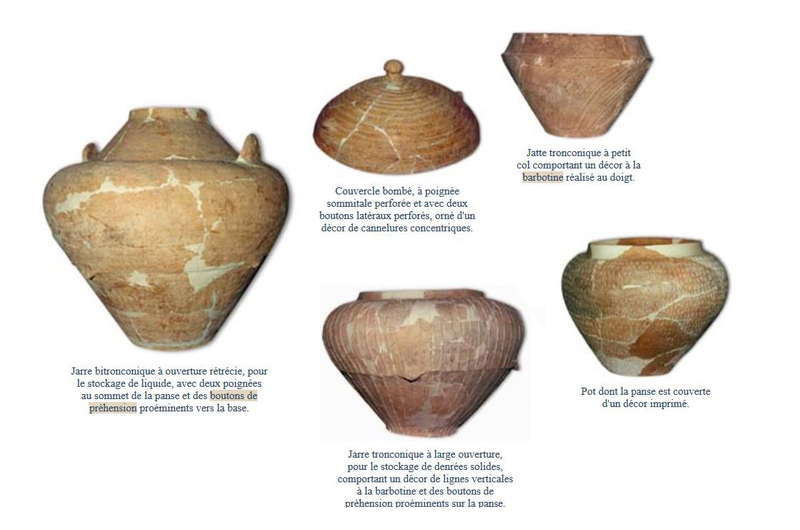The image features a collection of five ancient jars, distinctly depicted in individual photographs, accompanied by descriptive labels in French. These historical vessels exhibit a range of shapes and sizes, including traditional urn forms with wide openings approximately a foot in diameter. The collection contains various shades of brown, tan, and even some burgundy tones. The jars' surfaces are cracked yet well-preserved, highlighting their age and fragility. 

One of the jars resembles the top of a tandoori oven, while another has the natural flaking patterns akin to an onion's skin. A noteworthy jar includes geographic-like panels, reminiscent of country divisions on a map. Among the artifacts, there is also a lid that doesn't match the color of a nearby jar, suggesting they might not belong together. Other designs include an urn with rounded handles and one with a more angular, diamond-esque structure. These finely detailed and breakable pottery pieces suggest they are museum-worthy treasures, encapsulating the intricate craftsmanship of their era.